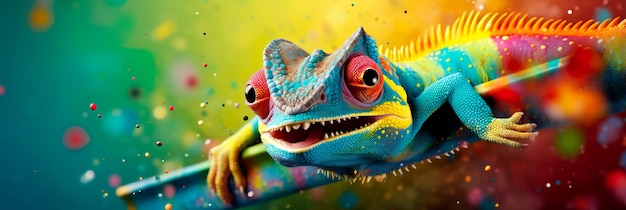The image depicts a highly colorful, computer-generated lizard, possibly a Gila monster or chameleon, positioned centrally with its head in the middle and body extending off the right edge. The lizard boasts a vivid, rainbow palette, featuring a blue head with pink splotches, red eyes with black centers, and a mouth slightly open to reveal tiny, pointy teeth. Its front legs are blue, transitioning to red and yellow with yellow feet, and its body transitions from blue to yellow along its spine, ending in a primarily red tail. Thin spines adorn the upper part of its body. The lizard appears to be resting on the edge of a surface, likely a metal tray or painted table covered in a myriad of colors. The background is a blurred, multicolored gradient starting with blue-green on the left, blending into splotches of yellow, blue, and red, and transitioning to blurry red with gray and purple spots on the right. The overall effect is a vivid and striking composition, rich in color and detail.